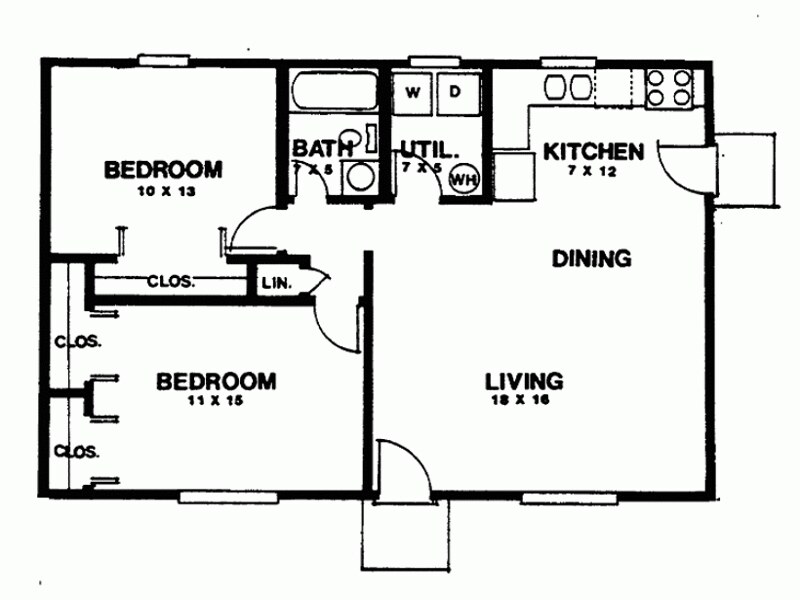This detailed floor plan illustration depicts a spacious, two-bedroom unit. The layout is represented schematically and is wider than it is tall. In the lower left-hand quarter, the main bedroom measures 11 by 15 feet and includes two generous walk-in closets. Adjacent to the main bedroom is a linen closet and a doorway leading to the primary bathroom, situated directly above the bedroom.

The second bedroom is positioned above the primary bedroom, completing the left-hand side of the unit. This arrangement hints that the plan could be for either an apartment or a ranch-style house. 

To the right of the master bedroom wall is the front door, which opens into a combined living and dining area, measuring 18 by 16 feet. This expansive space flows seamlessly into the well-appointed kitchen, which spans 7 by 12 feet and features an L-shaped counter with a double sink and a range. 

Beyond the living room, directly forward from the front entrance, lies a utility closet housing a washer and dryer, labeled "WD," and a water heater, labeled "WH." Additionally, there is a doorway off the kitchen, enhancing the unit's functionality and accessibility. This thoughtfully designed floor plan maximizes both comfort and practicality for its inhabitants.